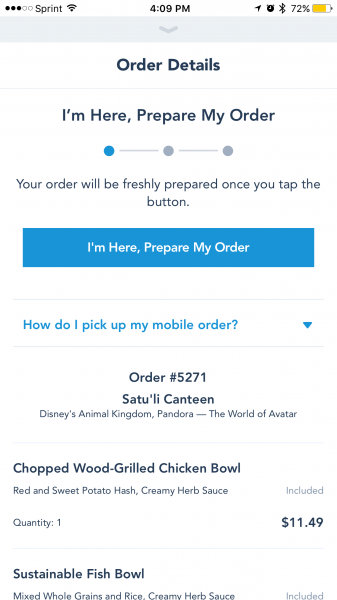**Image Description:**

Set against a solid white background, the image features a screenshot with multiple elements that provide detailed information about an order from Setouli Canteen in Disney's Animal Kingdom, Pandora, The World of Avatar. 

- **Top-Left Corner:**  
  - **Reception and Service Icons:** Three out of five circles indicating signal reception strength.
  - **Carrier Information:** "SPRINT" text along with a Wi-Fi icon.
 
- **Center Top:**  
  - **Time:** 4:09 PM.
  - **Battery Icon:** Showing 72 percent battery level.

- **Below Center-Top:**  
  - **Notification Bar:** Gray with a pull-down arrow icon.

- **Main Content Area:**
  - **Title:** ORDER DETAILS in bold black text.
  - **Status:** "I'm here, prepare my order," is shown beneath the title.
  - **Order Status Indicator:** A blue circle highlighted out of three possible circles.
  - **Instruction:** "Your order will be freshly prepared once you tap the button."
  - **Action Button:** A blue button labeled "I'm here, prepare my order."

- **Order Information:**
  - **Order Number:** 5271.
  - **Location:** Setouli Canteen, Disney's Animal Kingdom, Pandora, The World of Avatar.
  - **Menu Item:** Chopped wood-grilled chicken bowl.
  - **Price:** $11.49.